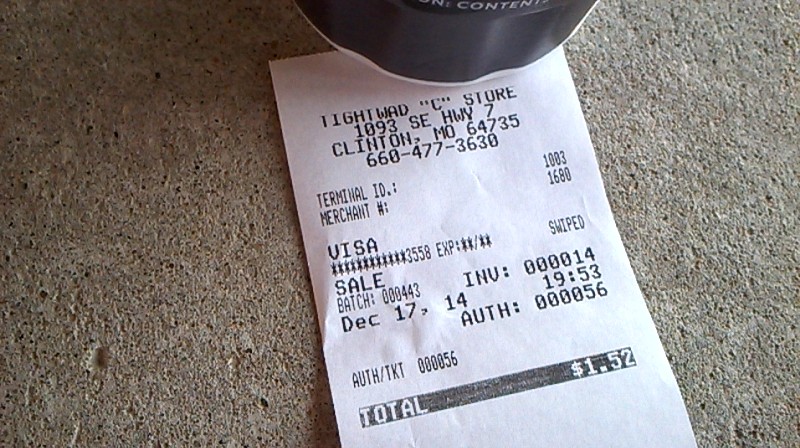This image captures a detailed shot of a receipt from Tightwad C Store, located at 1093 SE Highway 7 in Clinton, MO. The store's contact number is prominently displayed at the top in black ink. The receipt, printed in black ink on white paper, is photographed at an angle, extending from the lower right side of the frame towards the upper center. It rests on a gray, stone-like countertop, suggesting a concrete surface rather than fabric. To secure the receipt in place, a blue cylindrical object is positioned on top. The receipt details a Visa transaction amounting to $1.52, dated December 17th, 2014, and timestamped at 19:53.